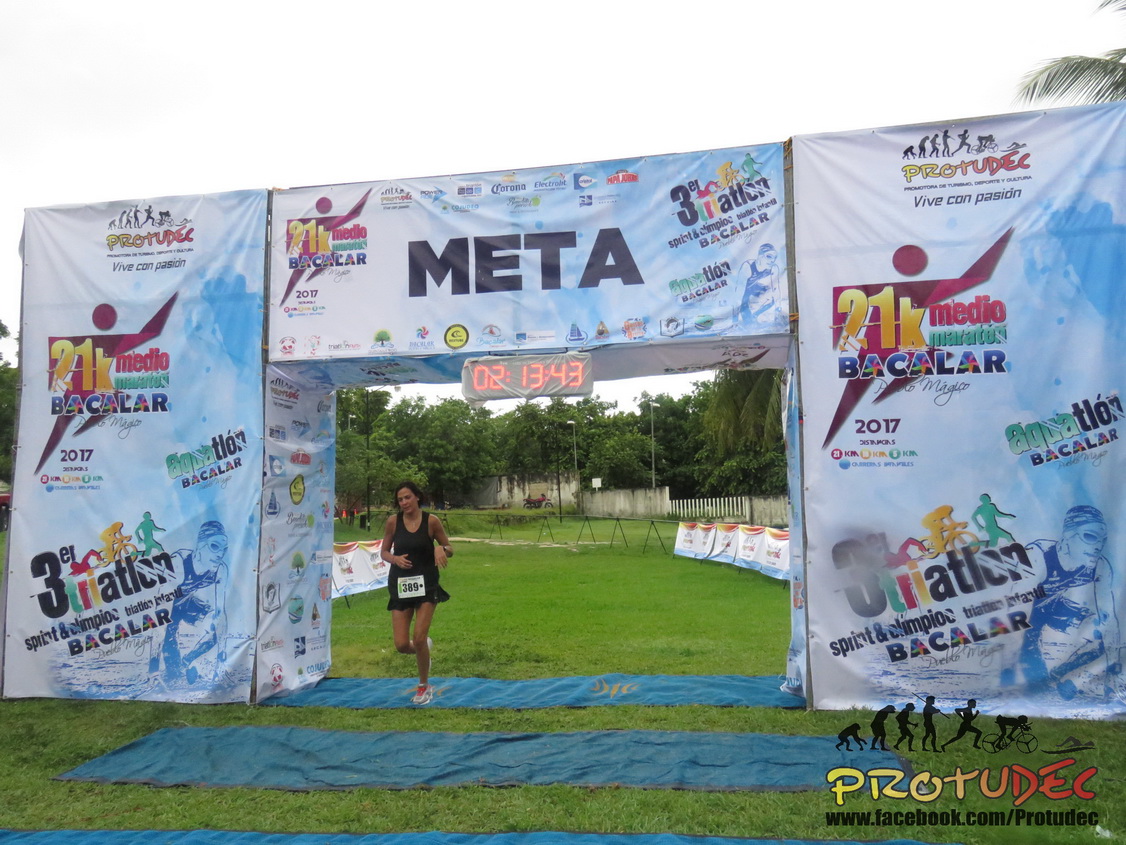This detailed image captures an outdoor race scene featuring a female runner with dark hair, dressed in a black tank top, black skirt, and white shoes with red laces. She wears a race number "389" pinned to the front of her attire. The runner is depicted just as she is crossing the finish line, marked by a rectangular archway with a banner labeled "Meta," and a large digital timer displaying her finish time of 2:13:43. The backdrop includes black, yellow, and red lettering advertising the 21K media bachelor event, indicative of an aquathon. Blue tarps are laid out on the ground beneath her, and a white fence and house are visible in the background, accompanied by a white sky and the fronds of a couple of palm trees. The bottom right of the image features the branding "PROTUDEC" and its Facebook link, alongside an evolutionary silhouettes graphic that transitions from ape to a human running, bicycling, and swimming.